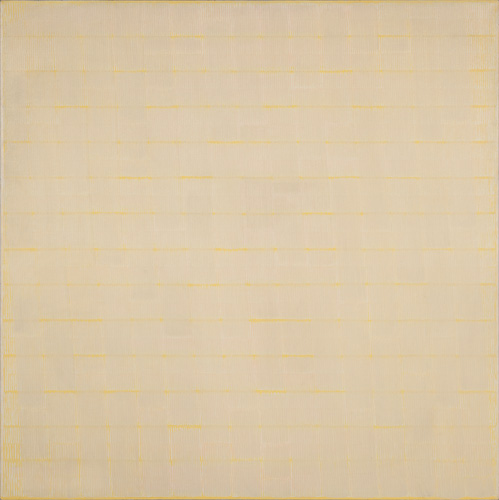The image is a close-up shot of a notepad paper fragment that appears slightly aged, with a white color tinged with yellow. The paper features light horizontal yellow lines running straight across, and due to the extreme zoom, only a small segment of the notepad is visible. The overall appearance is minimalistic and abstract, reminiscent of the minimalist art style, particularly resembling James Bishop's "Closed" from 1974. The backdrop is mostly cream-colored, and no other objects or details are present, giving it a simplistic and serene aesthetic.